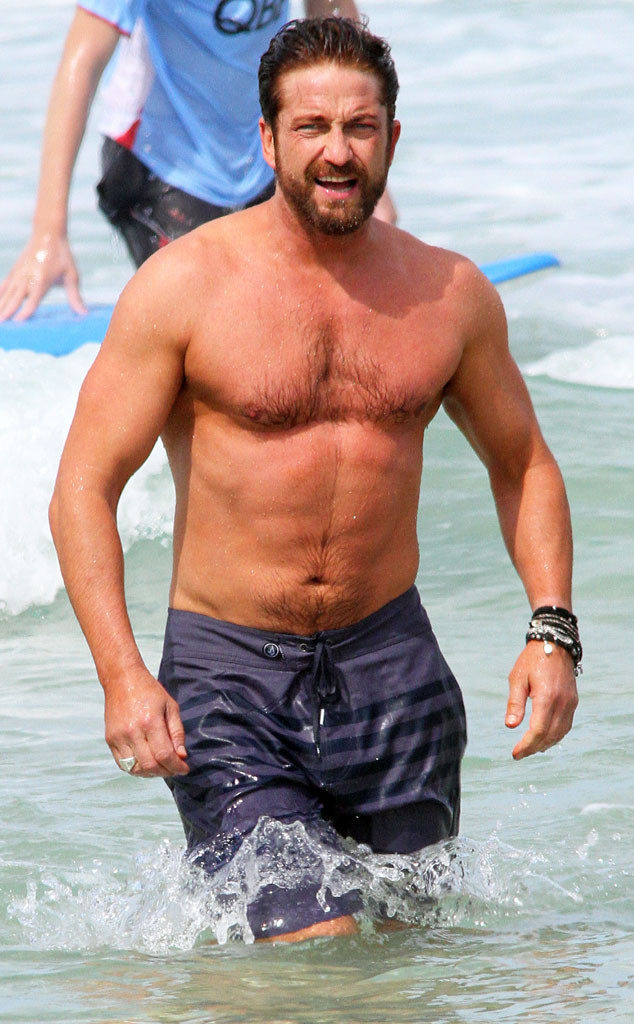In this dynamic beach scene, we see actor Gerard Butler emerging from a relatively shallow, clear body of water, with waves gently lapping around him. Wearing a deep purple swimsuit adorned with darker blue stripes, Gerard stands proudly at the center of the image, shirtless and with his tan skin glistening in the daylight. His hair is wet and slicked back, matching his damp beard, and he exudes confidence with a broad smile directed at the camera. A notable array of bracelets adorns his right wrist, alongside a ring on his right ring finger. Further enriching the composition, another individual is positioned at the top part of the image, wearing a blue shirt and black shorts, and appears to be getting onto a floating surfboard or pad. The beach setting is painted in vibrant hues of green, white, black, gray, tan, light blue, and red, all under a bright, midday sky. The image radiates a lively, sun-soaked atmosphere, capturing a joyful moment of leisure and splashing water.